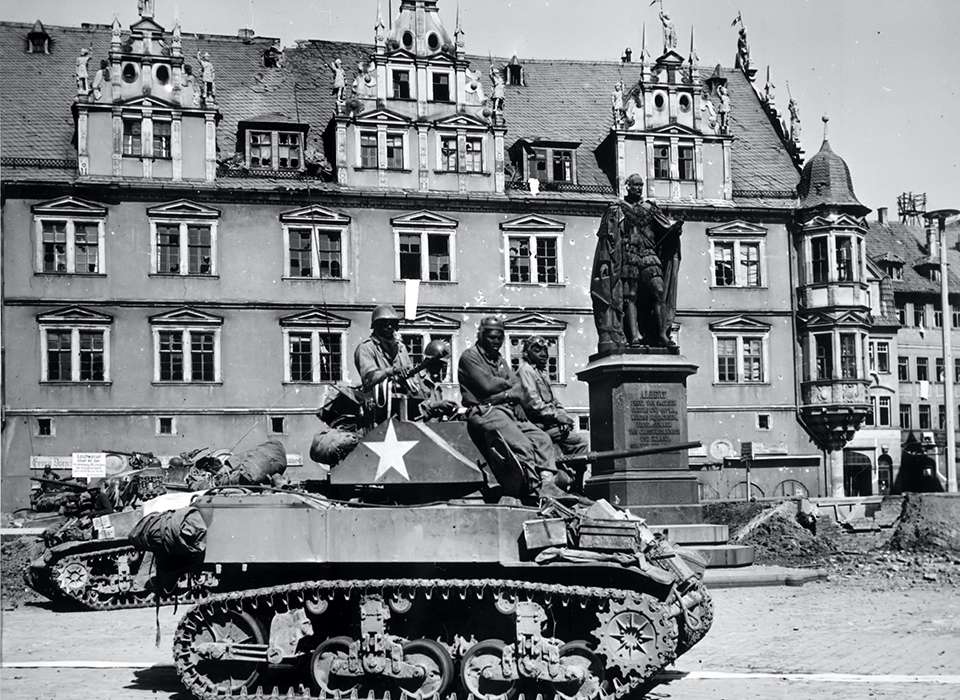This black and white photograph captures a moment from what appears to be the end of World War II, possibly in France. The focal point of the image is an American tank navigating through a street in front of a grand, albeit damaged, mansion. The tank, smaller by modern standards, carries approximately four to six soldiers. The vehicle is painted a grayish color with a prominent white star on its side and features visible treads and gears.

The tank is moving left to right in the frame, with its barrel pointed to the left. One soldier is emerging from the top hatch, wearing a helmet and a long shirt, while two other soldiers lean against the front, facing the camera. Another tank, barely visible, rolls off to the left, showing only parts of its structure.

The imposing mansion behind the tank stretches three stories high, with a slanted roof and multiple fixtures that appear to be additional rooms. The building has numerous windows, though its facade and roof show significant damage, possibly from bombings or gunfire, indicating the ravages of war.

In front of the mansion stands a tall statue of a man in a cloak and frilly shorts. The dark statue dominates the foreground, rising slightly higher than the tank. The photograph conveys a juxtaposition of war and refined architecture, hauntingly illustrating the impact of conflict on a once-elegant estate.